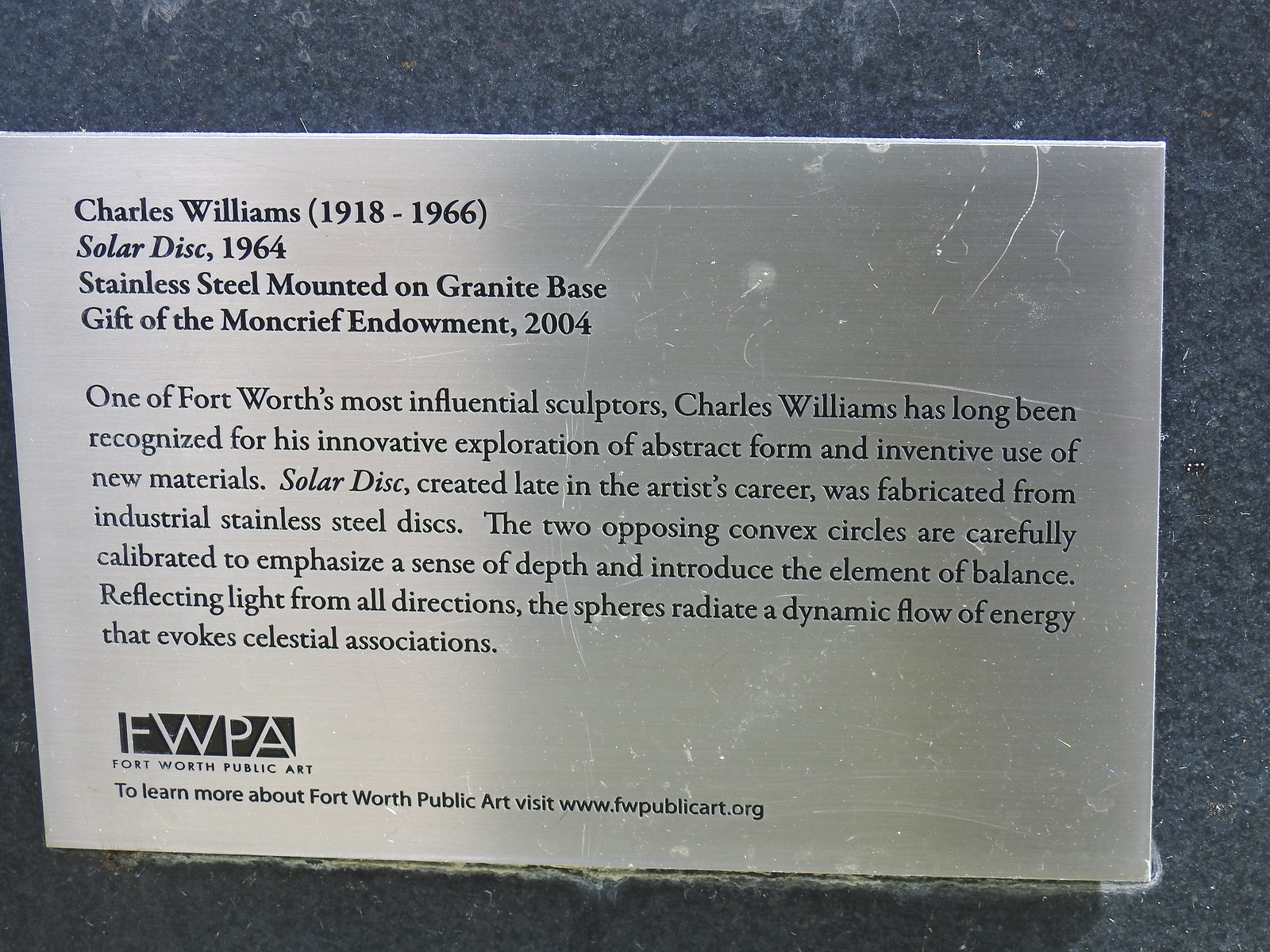This detailed color photograph showcases a close-up of a rectangular, silver metal plaque mounted on a dark gray granite surface. The top left corner of the plaque reads "Charles Williams (1918-1966)" in black lettering. Below this, in italics, it states "Solar Disc, 1964," followed by the note "Stainless steel mounted on granite base" and "Gift of the Moncrief Endowment 2004." These inscriptions highlight important details about the artwork.

The plaque further describes, "One of Fort Worth's most influential sculptors, Charles Williams has long been recognized for his innovative exploration of abstract form and inventive use of new materials. 'Solar Disc,' created late in the artist's career, was fabricated from industrial stainless steel disks. The two opposing convex circles are carefully calibrated to emphasize a sense of depth and introduce the element of balance. Reflecting light from all directions, the spheres radiate a dynamic flow of energy that evokes celestial associations." This detailed description of the artwork, which is not visible in the photo, emphasizes the artist's significance and the plaque’s intent to inform viewers about the sculpture.

At the bottom of the plaque, the logo "FWPA" for Fort Worth Public Art is displayed in white letters against a black background. Below the logo, it reads, "To learn more about Fort Worth Public Art, visit www.fwpublicart.org."